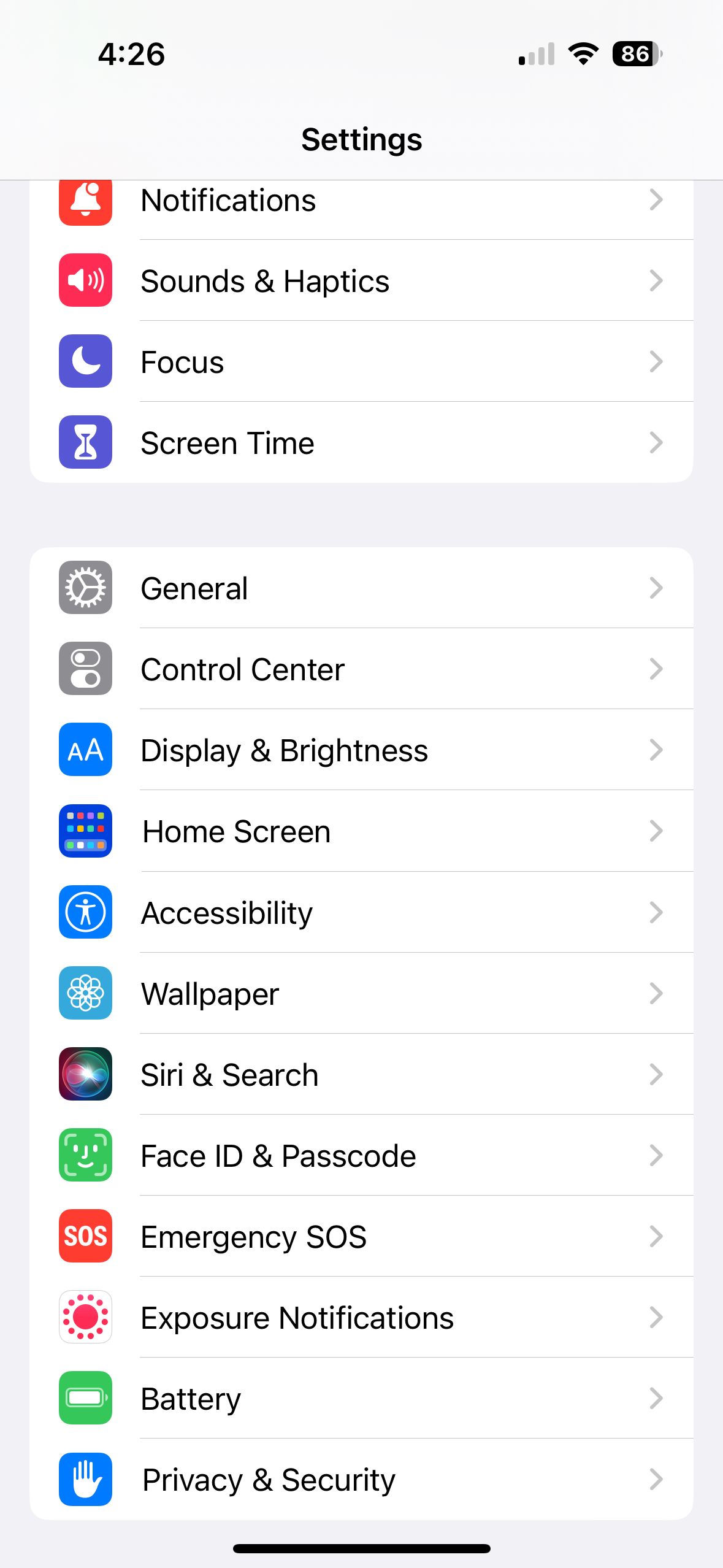The screenshot depicts a white background adorned with various colorful icons and black text. At the top, the number "426" is prominently displayed, followed by a Wi-Fi symbol resembling a funnel or tornado. To its right, there's a single signal strength bar and a battery icon showing 86% in white text on a black background.

Moving down, the word "Settings" appears in bold black text, separated by a gray line from the content below. The settings menu is neatly organized into white boxes with black text, each accompanied by a distinctive icon and a small arrow indicating more options.

1. **Notifications**: An orange box with a white bell icon.
2. **Sounds & Haptics**: A pink box with a white speaker icon.
3. **Focus**: A purple box with a white moon icon.
4. **Screen Time**: A purple box with a white hourglass icon.
5. **General**: A gray box with a white cogwheel icon.
6. **Control Center**: A gray box with several small white boxes icon.
7. **Display & Brightness**: A blue box with two white "A"s.
8. **Home Screen**: A blue box with colorful icons.
9. **Accessibility**: A blue box with a white person figure icon.
10. **Wallpaper**: A baby blue box with a flowery spiral white icon.
11. **Siri & Search**: A black background with a multicolored orb in pink, green, and blue.
12. **Face ID & Passcode**: A green box with a white abstract smiley face.
13. **Emergency SOS**: A red box with white "SOS."
14. **Exposure Notifications**: A white box with a pink circle icon.
15. **Battery**: A green box with a white battery icon.
16. **Privacy & Security**: A blue box with a white hand icon, palm out.

At the bottom of the image, a thin black line extends across the screen, marking the end of the settings list.